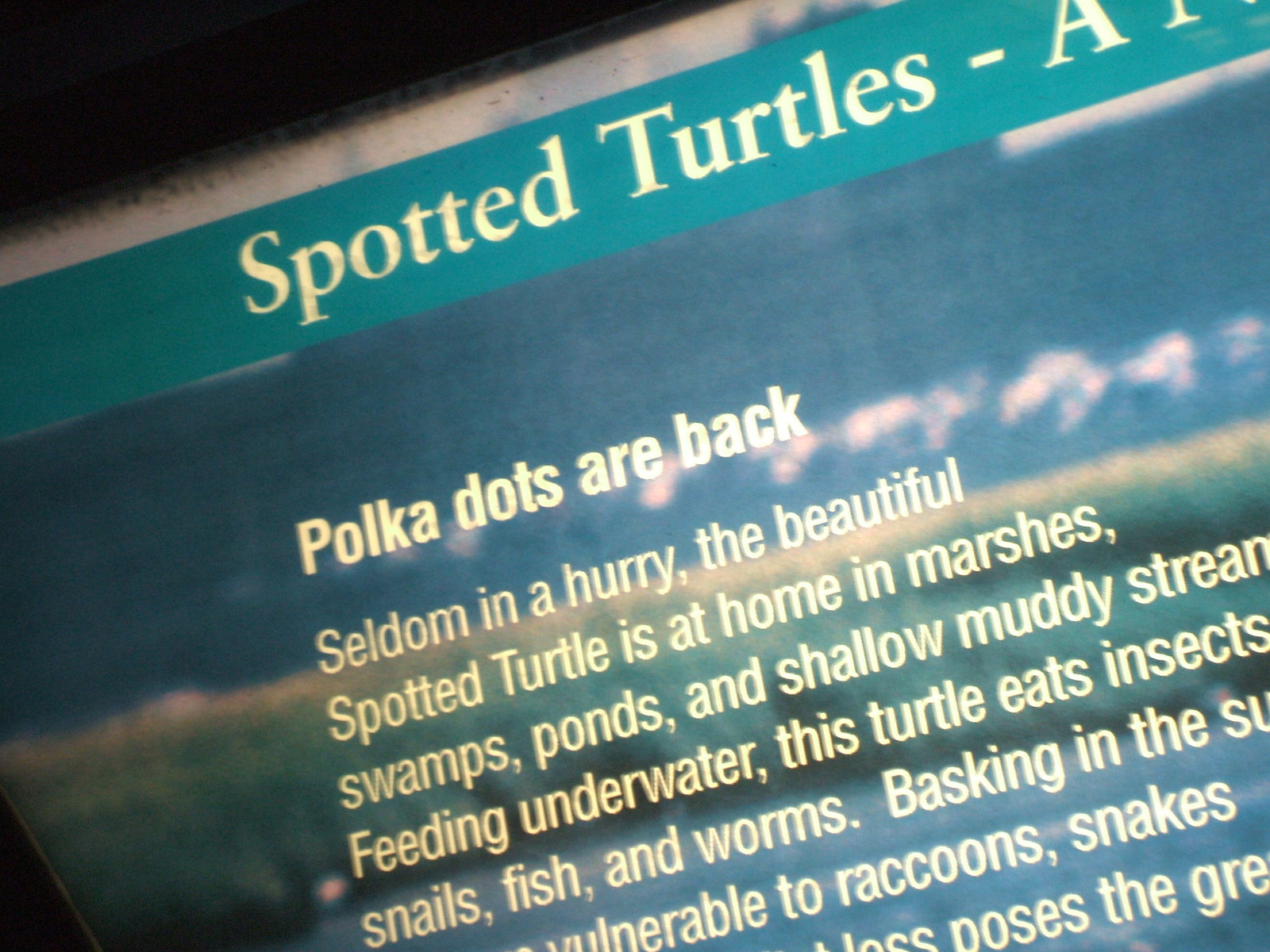This image appears to be a close-up photograph of a section of an informational webpage tilted counterclockwise, possibly taken from a laptop screen. The page features a combination of colors, including blue, green, white, and a little bit of yellow, with a faded background image of water and grass. At the top, in large white text against an aqua blue banner, are the words "Spotted Turtles." Below that, in smaller white text, it reads "Polka dots are back. Seldom in a hurry, the beautiful spotted turtle is at home in marshes, swamps, ponds, and shallow muddy streams. Feeding underwater, this turtle eats insects, snails, fish, and worms." The text is then cut off but includes phrases like "basking in the," "vulnerable to raccoons, snakes," and "poses the GRE." Additionally, the edges of the image reveal black areas, indicating the limitations of the photo's framing.